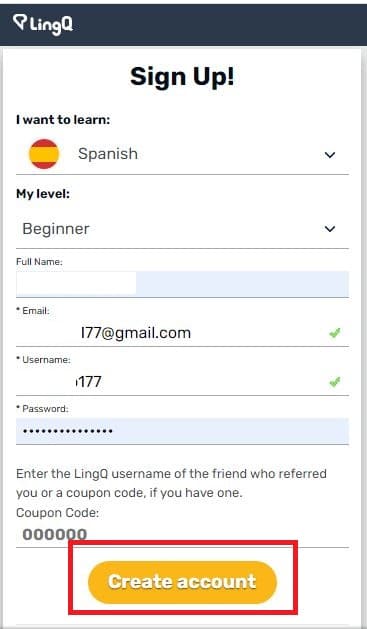The image features a sign-up form with several distinct sections. At the top, there is a blue rectangle featuring a small symbol and the text "LingQ" or "LingGo." Below this, the background transitions to white, with a light gray, outlined rectangle centrally displayed. Inside this rectangle, the text reads "Sign Up." 

Beneath the rectangle, there is a prompt stating "I want to learn." Next to this, a circular icon is divided into three horizontal sections—red on the top and bottom, and yellow in the middle—with the word "Spanish" inside. To the right of this icon, an arrow points downward next to the text "My Level," which indicates "Beginner" with another downward-pointing arrow beside it.

Further down, there are fields for "Full Name" (with the content whited out) and "Email," which is followed by a green check mark indicating a valid entry. Below these fields, there are sections for "Username" (also whited out) and "Password," represented by a series of dots. 

There is an additional prompt requesting the "LingGo username of the friend who referred you or a coupon code if you have one," followed by a field labeled "Coupon Code," pre-filled with “000000.” 

At the bottom of the form, a rectangular red button features the text "Create Account," colored in an orangey-yellow hue with rounded edges.